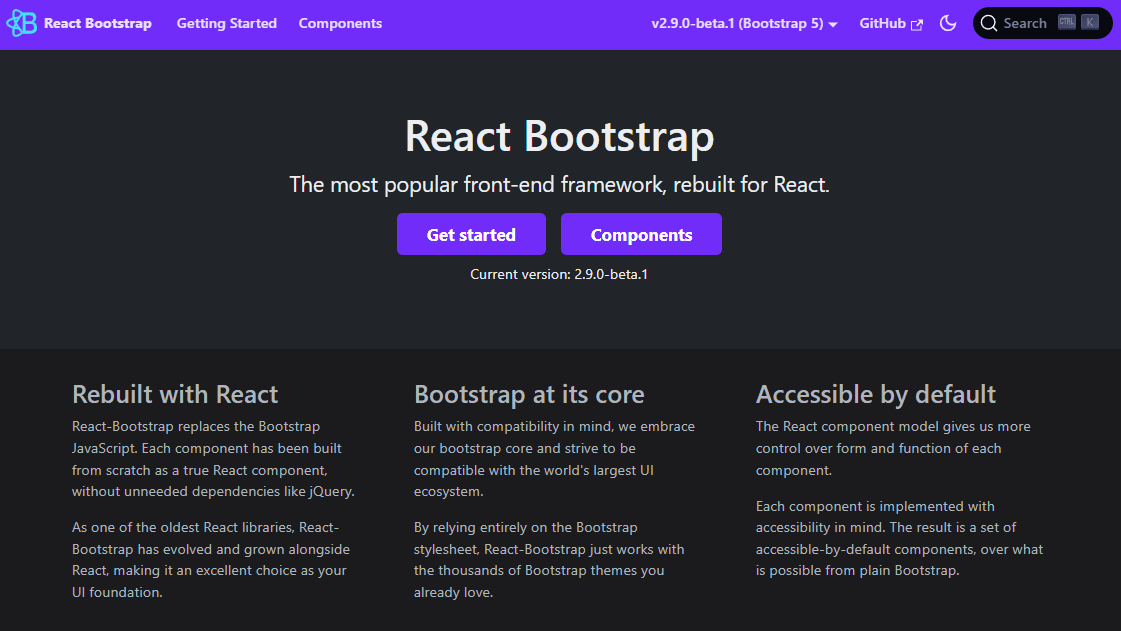This screenshot captures a webpage focused on React Bootstrap. In the top left corner, the header reads "React Bootstrap: Getting Started and Components." The top right corner features a "Beta" label, a "Bootstrap 5" tag, and a search bar. Below this header section, the page has a black background with white text.

The main content showcases an enlarged title, "React Bootstrap" followed by the tagline, "The most popular front-end framework rebuilt for React." Directly beneath this tagline are two prominent buttons: "Get Started" and "Components." The current version listed is "2.9.0 Beta.1."

The content is divided into three descriptive columns:

1. **Rebuilt with React:** This section explains that React Bootstrap replaces the traditional Bootstrap JavaScript. Each component is meticulously redesigned as a pure React component, eliminating unnecessary dependencies like jQuery.

2. **Bootstrap at its Core:** Emphasizing compatibility, this section highlights the project’s commitment to maintaining Bootstrap's core principles. The goal is to remain in harmony with the world's largest UI ecosystem.

3. **Accessible by Default:** Here, the focus is on accessibility. The React component model provides greater control over each component's form and function, ensuring they are accessible by default—surpassing the accessibility capabilities of standard Bootstrap.

This structured layout summarizes the offerings and benefits of React Bootstrap, concluding the webpage.